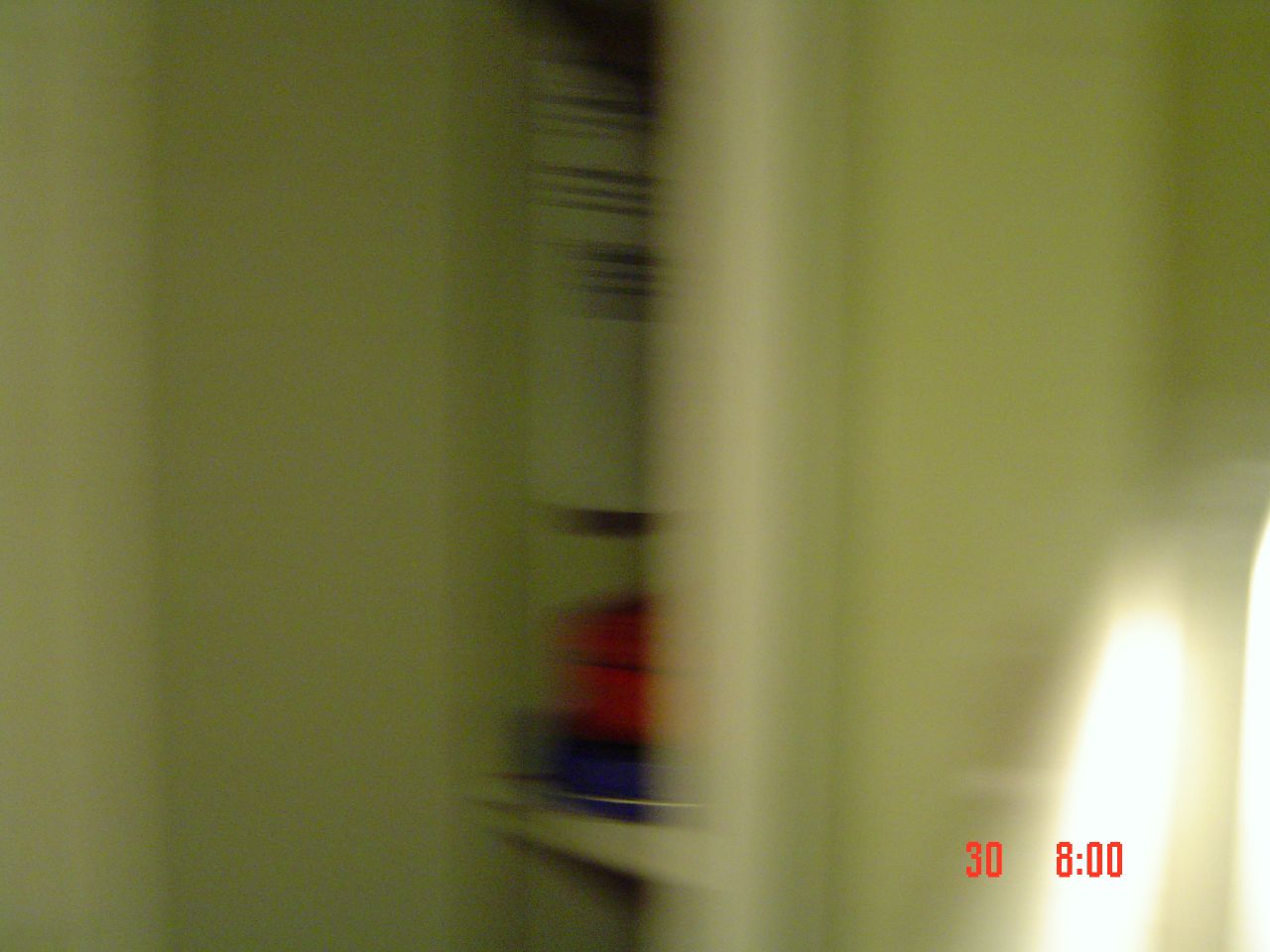A hastily taken, extremely blurred photograph featuring an overexposed and washed-out white kitchen scene. The right side of the image showcases a white fridge freezer, its edges fading into the equally white background. The fridge door is open, revealing red and blue items in the door's shelves. The scene is dominated by varying shades of whites and beiges, depending on the lighting. On the left side of the frame, a cluttered shelving system or cabinet is visible with several shelves. The middle shelf holds a blue pan or plate with a red container on top, and what appears to be dish towels hanging inside, one plain white and one striped white with gray. The left side also has a wall with some brown lines or wainscoting. The photo includes a portion of a brighter, possibly yellow-beige wall and an open doorway, revealing more shelving inside. There is also a printed red text at the bottom reading "308:00." The entire image appears overexposed, blurred with trailing effect, likely due to the camera moving while capturing the scene.